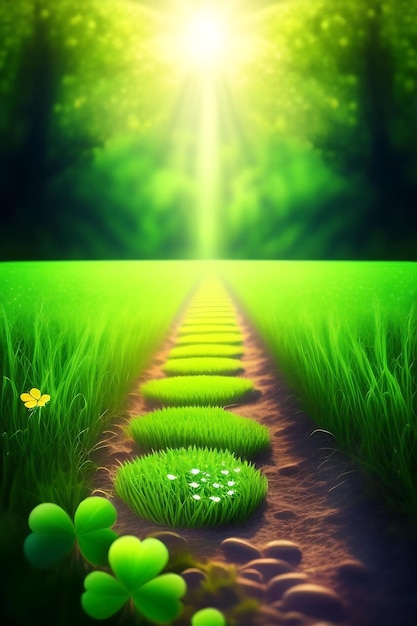The image features a surreal, possibly computer-generated, landscape divided into two distinct panels. The upper section is dominated by a blindingly bright white light that appears to emanate from the middle, casting its glow downward. Surrounding this central light is a gradient of vibrant, almost neon green that gradually deepens towards the edges, eventually merging into an almost black hue before transitioning back to darker shades of green. The top half of the image evokes a forest-like scene with sunlight filtering through, creating a dreamlike, slightly blurred effect.

The lower section displays a fantasy-like green field. A central path made of circular patches of grass stretches infinitely into the distance, flanked by taller grass on either side. The path appears to be covered in hay-like dead grass, contrasting with the vivid green surrounding it. In the foreground, small clovers dot the scene, particularly noticeable in the lower left-hand corner. To the left side of the path, a small yellow five-petal flower stands amidst the grass, while the first circular grass patch along the path features a few delicate white flowers. The entire scene is framed by the lush, almost luminescent green of the grasses, enhancing the surreal and vibrant quality of the image.